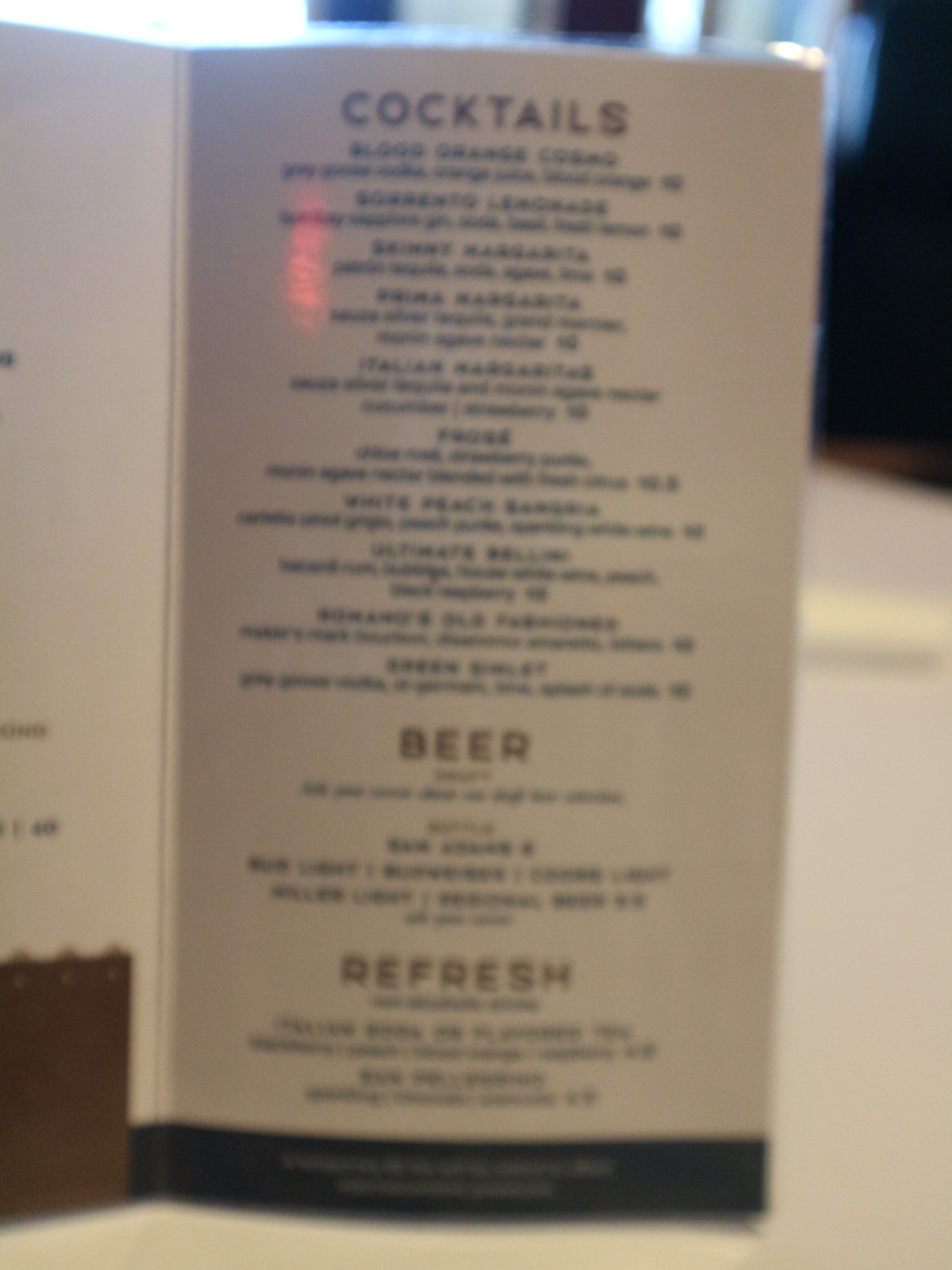This is a vertical, close-up image of a slightly blurred menu listing alcoholic beverages. The menu is printed on a stiff, likely coated, paper that is positioned upright as if being held for viewing. The contents are laid out from top to bottom, starting with a list of available cocktails and their prices. This section, occupying a little over half of the menu, is followed by a shorter list of beers. Below the beer section, there is a category labeled "Refresh." A black bar spans across the bottom of the menu. The headers are in a dark brownish hue, while the descriptions of the drinks and their prices are in black ink. The background shows a white or off-white tablecloth, adding a subtle contrast to the overall image.